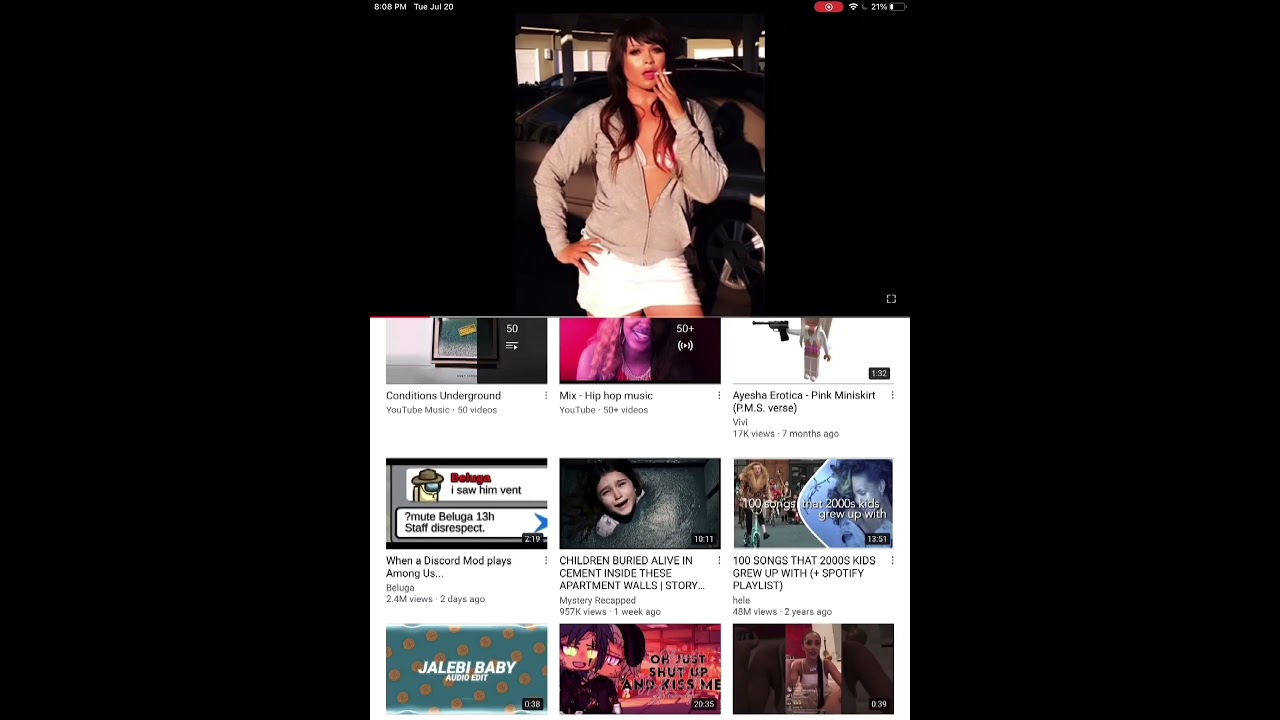The image captures a paused video playing on a website, set against an entirely black background. A mobile taskbar or notification center is visible across the top of the image. The video features a woman standing in a parking garage or similar parking area, with a vehicle seen behind her. She is dressed in a white skirt and a light gray zip-up jacket, and she has long brown hair. The woman is smoking a white cigarette, with her free hand resting on her right hip. Below the video frame, there is a white box displaying a selection of video thumbnails arranged in three rows, each containing three tiles.